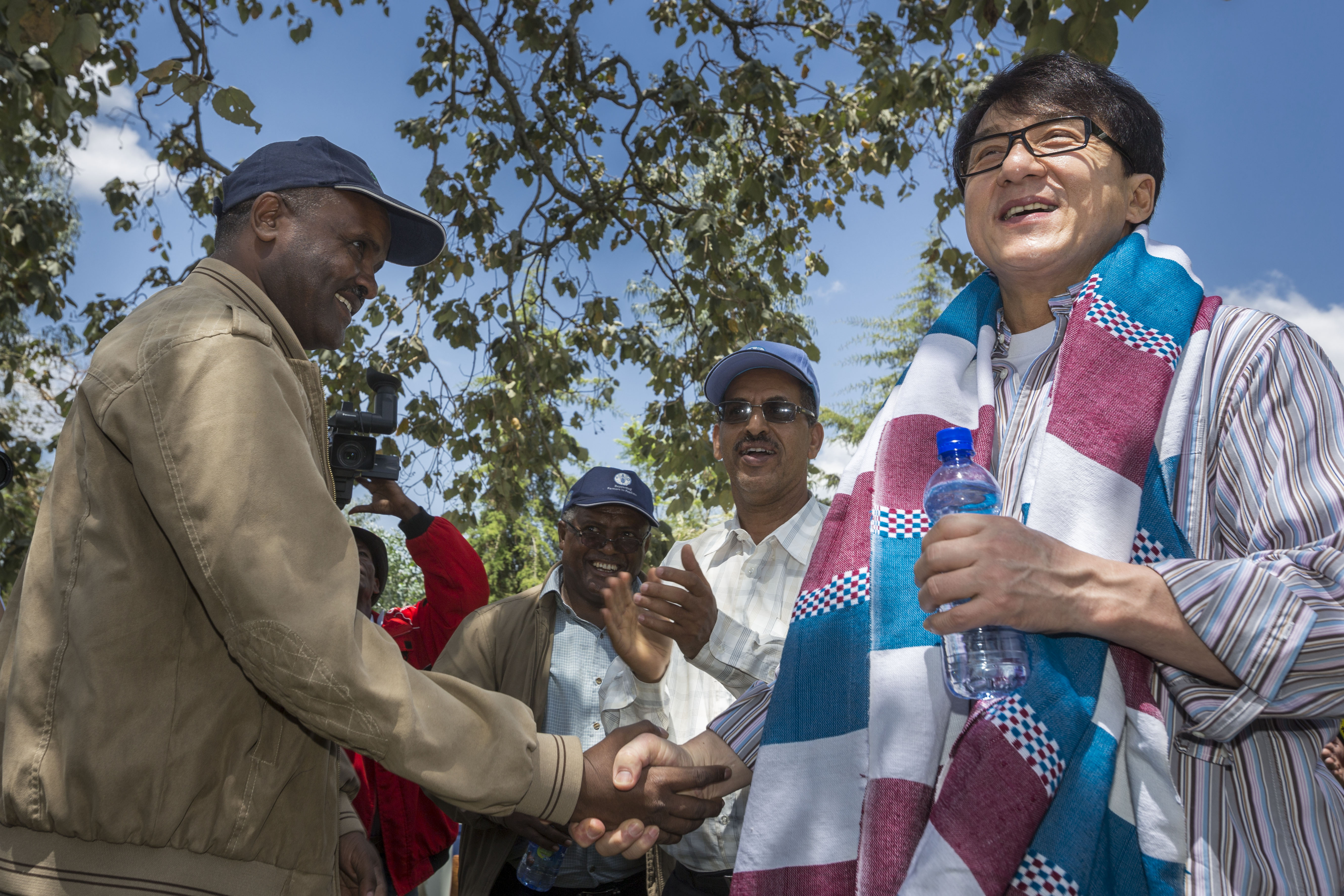The photograph captures a lively outdoor scene under a large tree on a bright, sunny day with a clear blue sky. Prominently featured on the right side is the renowned martial artist and actor Jackie Chan. He is smiling warmly as he shakes hands with an African-American man in a tan jacket and a navy blue baseball cap. Jackie Chan holds a water bottle in his left hand and wears black-rimmed glasses, with a shawl draped over his neck. The shawl is adorned with solid blocks and checkered patterns in pink, blue, and white hues. His shirt is shirt striped with an array of colors, including white, light blue, brown, and dark blue.

In the background, slightly out of focus, are three men. One of them holds a camera or camcorder, capturing the moment, while the other two, both wearing baseball caps, applaud and smile at the handshake. The scene conveys a casual yet potentially professionally captured moment, possibly from a fan meet-and-greet event, enhanced by the diverse, vivid colors of the environment and the attire of the individuals present.